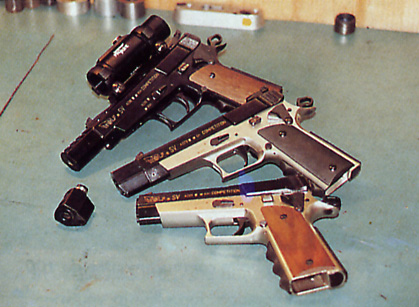On a gray, slightly blue-tinted metal tabletop, three distinct heavy-duty handguns are arranged in an arc, with their barrels pointing toward the bottom left corner, and the handles oriented toward the upper right. Each gun showcases different characteristics and materials.

The top gun, notably equipped with a scope and what appears to be a silencer or compensator, has a light wooden grip and an entirely black barrel with blurry white or gold writing on the scope. 

The middle firearm features a dark wooden inset on a silver handle, with a black slide and additional metal at the front. This gun appears to have a unique blue area running along the top and the front of the barrel.

The bottom pistol displays a lighter wooden handle with a black top and silver base, accompanied by gold letters near the barrel. A separate attachment lies next to it. 

The backdrop includes various small metallic objects, likely gun-related components, with one appearing cylindrical and another more oblong. Together, these elements form a visually striking and meticulously detailed arrangement of firearms.